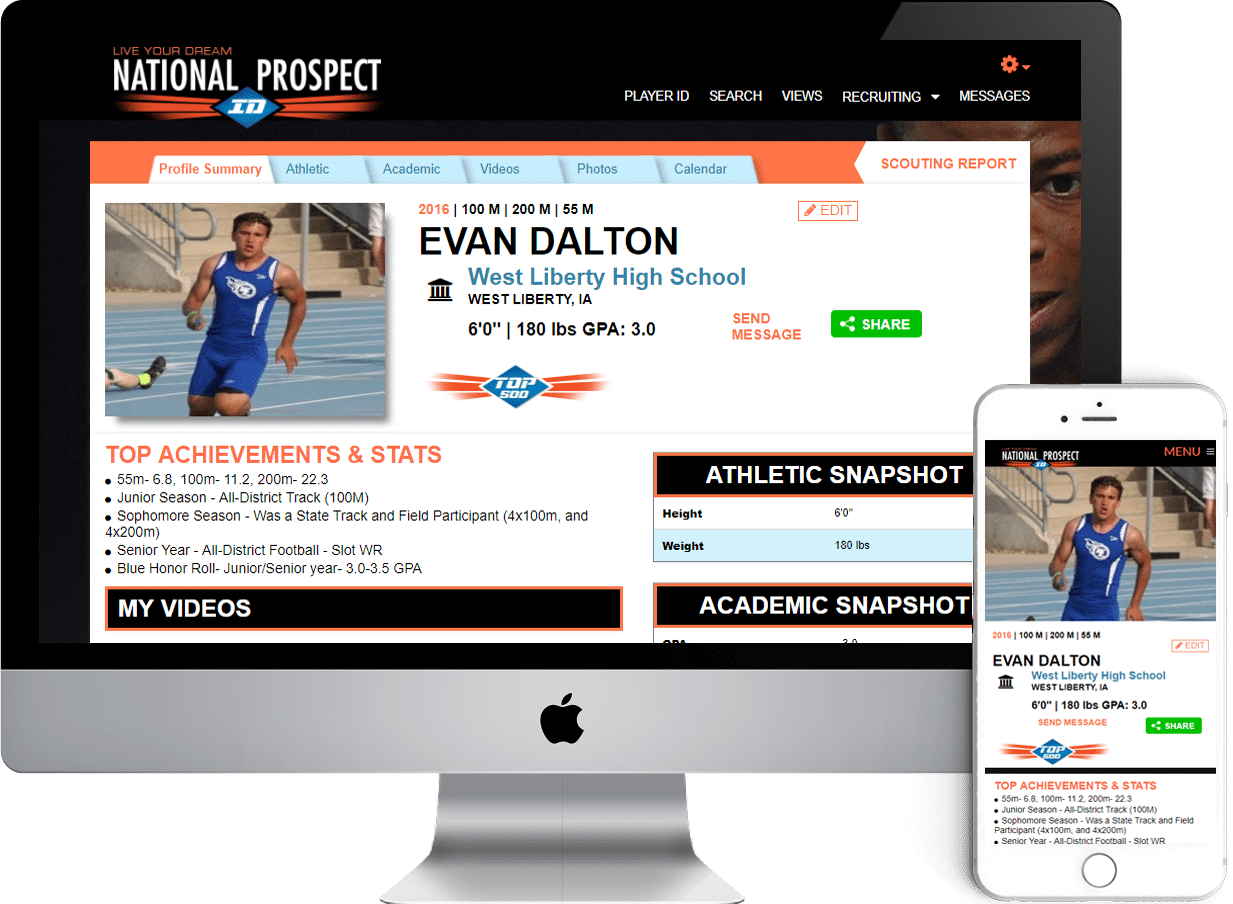In the image, a Mac computer and an iPhone are shown side-by-side, both displaying the same website—National Prospect ID. Prominent text on the website reads, "Live Your Dream." The computer screen reveals a navigation menu featuring options like Player ID, Search, Views, Recruiting, and Messages. Both devices display an image of a man running on a track. 

On the computer screen, additional details are visible, including sections labeled Profile Summary, Athletic, Academic, Videos, Photos, and Calendar. The profile belongs to Evan Dalton from West Liberty High School, listing his height as 6 feet, weight as 180 pounds, and GPA as 3.0. He is ranked in the top 500 athletes. 

Both the computer and phone display a list titled "Top Achievements and Stats." Exclusive to the computer screen are sections named My Videos, Athletic Snapshot, and Academic Snapshot.